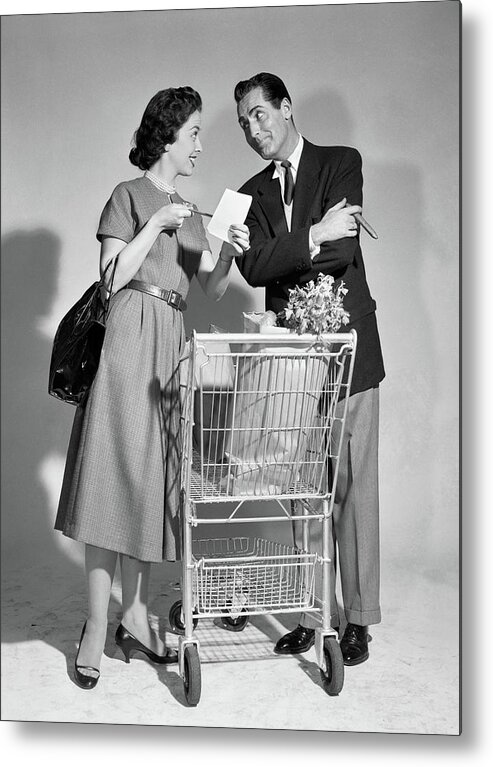This black and white photograph appears to depict a married couple engaging in a light-hearted discussion over a shopping list. Set against a flat background with their shadows cast prominently on the wall, the image captures a vintage mid-20th century atmosphere, likely from the 1960s. The woman, situated on the left, sports short, curly dark hair and dons a knee-length dress with a belt around her waist, complemented by a pair of high heels. A large black purse hangs from her elbow. She holds a piece of paper, presumably a shopping list, and points at it with a pen while looking at the man. The man, on the right, is dressed in a full suit with a tie and holds a cigar in his right hand. He has a smirk on his face as he listens to the woman. Between them stands a shopping cart containing groceries, including what looks like celery peeking out from a bag. Both individuals seem amused, smiling at each other, suggesting a candid, joyful moment. The spotlight effect casting their shadows gives the photograph a staged, possibly cinematic quality, hinting that they might be actors on a movie set.